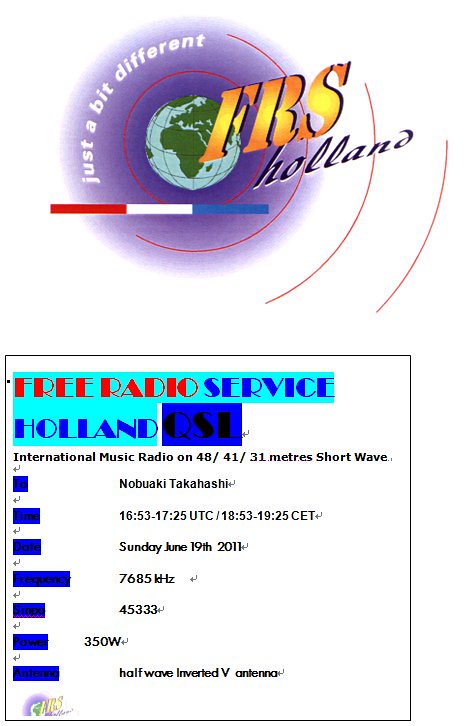The image is a digital flyer advertising a radio broadcast. The background is white, divided into two main sections. Dominating the top half is a globe rendered in a 2D cartoon style, focusing on Africa, with a surrounding purple cloud-like circle. Over the globe, bold capital letters "FRS" in a gradient of orange and yellow stand prominently, with the word "Holland" in cursive purple text just below.

Encircling the left side of the purple cloud are the words “just a bit different” written in white font, following the cloud's edge. Below the globe is a thin horizontal rectangle divided into thirds with colors red, white, and blue from left to right. Directly beneath this bar, there's a black-outlined square box with the words "Free Radio" in red, "Service" in blue, and “Holland” also in blue. Additionally, the letters "QSL" appear in black over a dark blue background.

In smaller text below these prominent elements are the details "International music radio on 48/41/31 meter shortwave." To the left, a list of somewhat obscured words appears in black text with a dark blue highlight. On the right, the list reads: "Nobakari Takahashi, Sunday, June 19th, 2011, 7685 kHz, 45333, 350W, half-wave inverted V antenna". There's also a symbol on the bottom left, seemingly saying "C US".